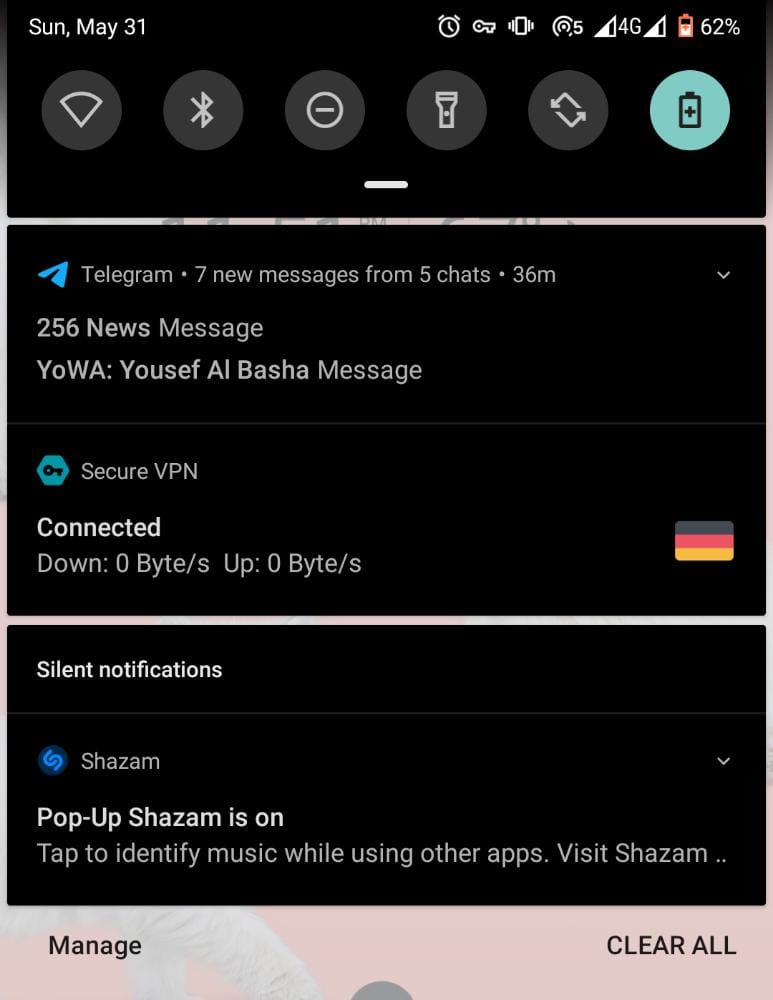**Detailed Description:**

The image displays a smartphone screen with various notifications and status indicators.

**Top Section:**
- **Date and Icons:** 
   - The top header shows "Sunday, May 31st."
   - An array of icons follows, including a reminder icon (alarm), a key icon for a secure app or feature, a vibrate icon, a "5G" icon (though marked just as "5"), and reception bars showing "4G" with three out of four bars filled.
   - Another reception icon also indicates three out of four bars, alongside an orange battery icon displaying "62%."
   - A Wi-Fi signal icon is present here as well.

Below the header are six circles against a black background, representing quick settings options:
   - Wi-Fi
   - Bluetooth
   - A straight bar (likely indicating signal strength or some connectivity feature)
   - Flashlight
   - Refresh
   - A battery meter

**Main Field:**
- The primary section of the screen shows a black field with app notifications and widgets:
   - **Telegram Notification:** Displays "70 messages from 5 chats, 36 minutes ago," and "256 new messages" along with a message from Yousef Al-Basha.
   - **Secure VPN:** Indicates that the VPN is connected with "0 bytes down" and "0 bytes up," including the German flag on the right side.
   - **Silent Notifications:** 
     - Shazam is mentioned here, showing "Pop-up Shazam is on. Tap to identify music while using other apps," along with "Visit Shazam dot dot..."

**Bottom Section:**
- There are two buttons at the bottom of the screen:
   - **Manage** on the left
   - **Clear All** on the right

**Icon Descriptions:**
- Each notification has corresponding small blue icons on the left:
   - The Telegram icon
   - The Secure VPN icon
   - The Shazam icon

These icons are reduced versions of their respective logos.

Overall, this screen shows a detailed and informative snapshot of the user's current notifications and status indicators, providing a comprehensive overview of ongoing tasks and connectivity details.